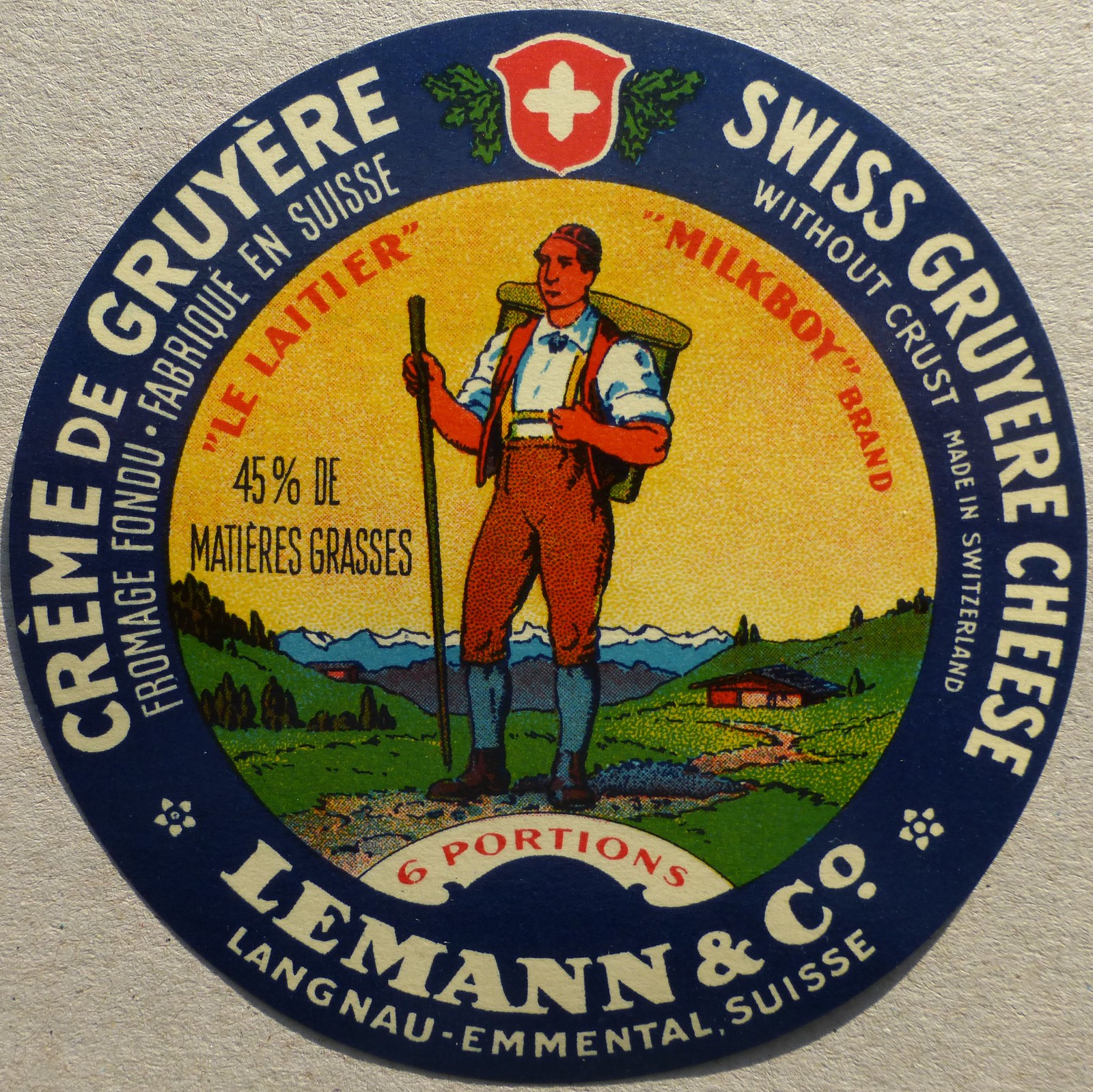The label is round with a dark blue border, featuring white lettering that reads "Crème de Gruyère fromage fondue fabrique en Suisse." It prominently displays a picture of a man dressed in traditional Swiss clothing, wearing knickers, suspenders, a white shirt, and blue socks. The man carries a square backpack on his back and holds a walking stick in his right hand. He stands on a patch of green ground, with a small house or barn to his left and mountains in the background. The central part of the label has a yellowish top. On the right side, the text reads "Swiss Gruyère cheese without crust made in Switzerland." At the bottom, the label states "Lehmann and Company Langnau-Emental Swiss." In addition, the label mentions "Le Laetitre Milk Boy brand 45% Metier grasses six portions" in red. The Swiss logo, a shield with a white cross surrounded by greenery, is also present. The entire label, which appears like a piece of paper affixed to the container, sits on a white stone surface.